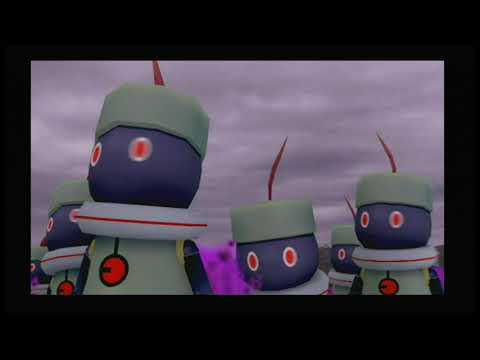This screen capture, possibly from a child's cartoon or an internet show, presents a pixelated and slightly shrunken image with a black border surrounding it. The setting is outdoors under an overcast sky, suggesting impending rain. The scene features six identical, non-human characters standing side by side in a nearly square, horizontal rectangle frame. These characters have round, blue faces with large, red eyes encircled by white. They lack visible noses or mouths, contributing to their robot-like appearance. Each character wears a cylindrical, gray cap resembling a vintage airliner stewardess hat from the 60s, adorned with a red antenna. Additionally, they have a white donut-shaped accessory with a red stripe around their necks and wear matching gray vests with a prominent red circle centered by a black border on their chests. These vests are complemented by purple sleeves, adding a colorful contrast to the overcast background. The overall effect suggests they might be puppets from a strange, whimsical children’s show, their eerie uniformity and unusual attire creating a visually striking and memorable image.